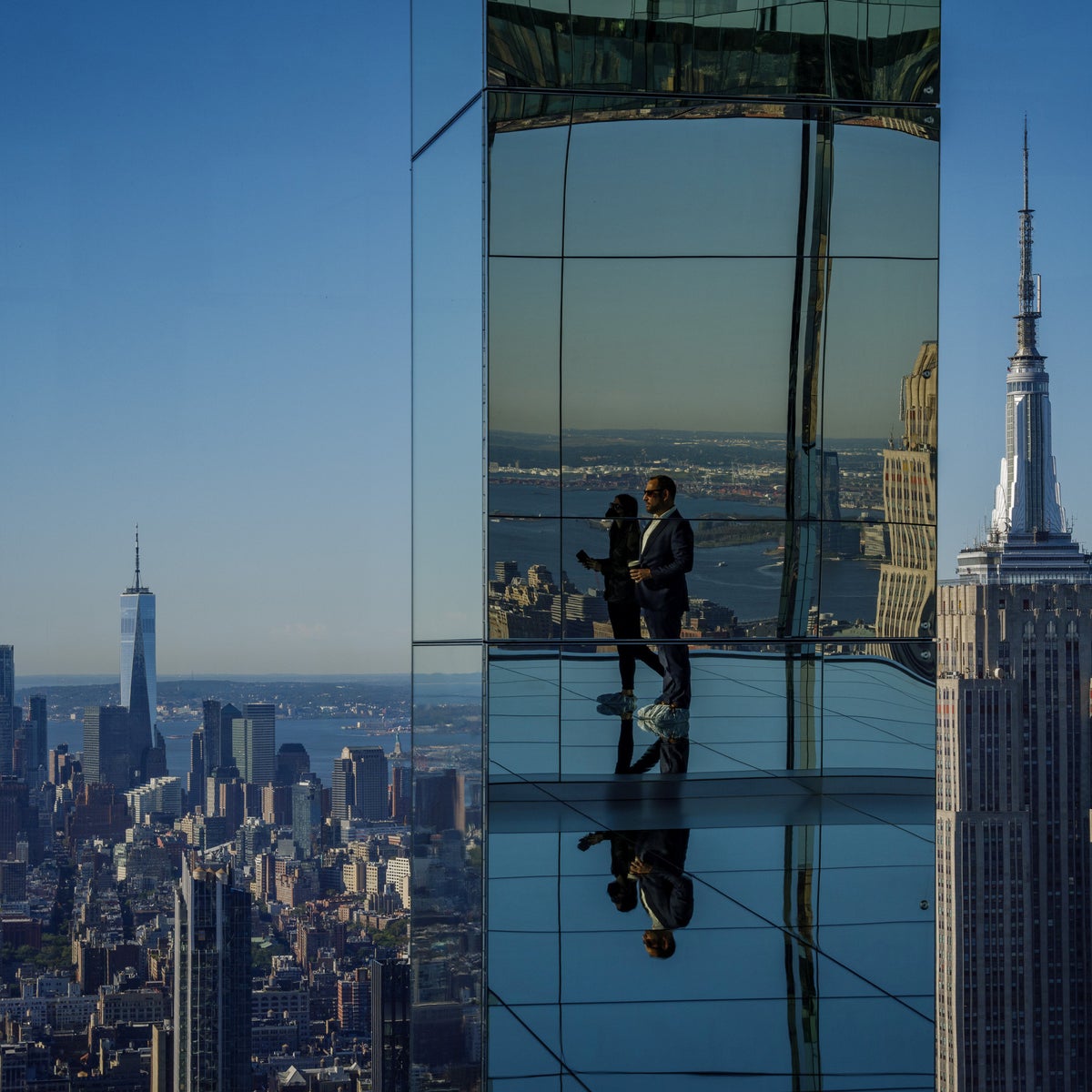The photograph captures a complex and intriguing scene featuring a tall, metallic skyscraper with a highly reflective exterior, likely situated in a major city such as Manhattan. Prominently reflected on the side of this building are two individuals, resembling a man and a woman, both dressed in business attire— the man is specifically noted to be wearing a white shirt, black suit, and black sunglasses. They are standing on what appears to be a glass or mirror-like tiled floor, further contributing to the surreal quality of the image. The individuals exude a prestigious aura and are gazing off to the left, seemingly overlooking the expansive city skyline. The backdrop showcases a range of predominantly rectangular buildings in neutral colors like silver and gray, with numerous windows. The sky above transitions from a dark blue near the top to a lighter blue as it meets the horizon, indicating that it might be midday or approaching dusk. The overall setting includes other notable city features, such as the river in the background and a variety of skyscrapers, with most of the image dominated by the expansive blue sky.